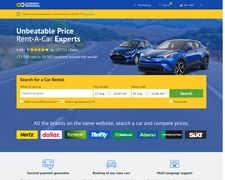Screenshot of a Car Rental Website:

The screenshot captures the homepage of a car rental website, though the text is primarily blurry and challenging to discern. 

- **Top Left Corner**: Features an unreadable logo.
- **Background**: A blue background extends across the top of the page, with additional illegible text.
- **Border**: Immediately below the background image is an orangish-yellow border with more unreadable text.
- **Main Photo**: Dominating the page is a photograph of two blue cars side by side—a prominent SUV in the foreground and a smaller vehicle in the background. They are situated on a winding road, likely in a rural area with potential mountains and farmland in the distance, though the image is also somewhat out of focus.
- **Text on Left Side**: Clear text reads, "Unbeatable Price Rental Car Experts," accompanied by a star rating that seems to fall between 4 and 5 stars, though additional text in this area remains blurred.
- **Search Section**: Beneath the photo is a large box with an orange background containing the text, "Search for a Car Rental." This section includes various option boxes, but their text is too blurred to read.
- **Logos for Companies**: Notable logos for Hertz and Thrifty are visible among other indistinct company logos.
- **Bottom Icons**: Additional icons are present at the bottom of the page, including one of a vehicle and another that might represent a telephone.

This detailed description should help in imagining the content and layout of the blurred screenshot.